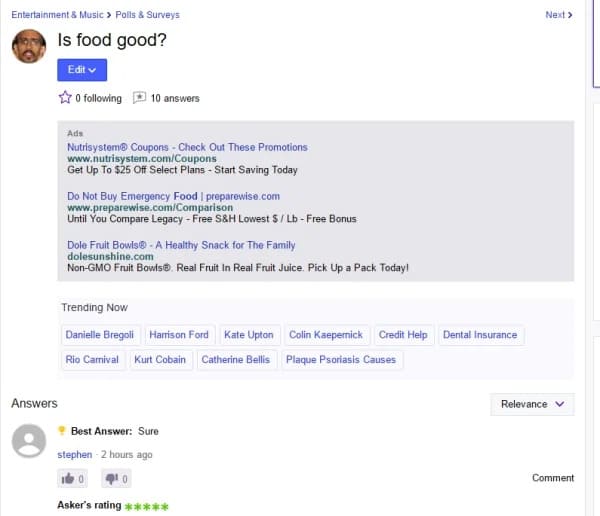The image displays a multifaceted interface divided into different sections. 

In the top-left corner, there are categories labeled "Entertainment and Music" as well as "Polls and Surveys." Underneath, the question "Is food good?" is posed, followed by a blue square that says "Edit." It shows that there are 0 followers and 10 answers.

A central segment advertises NutriSystem coupons with a promotion directing viewers to visit www.nutriSystem.com/coupons to get up to 24% off and $25 off select plans for immediate savings. Another advertisement warns against buying emergency food from preparewise.com and suggests comparing options at www.preparewise.com, highlighting "Legacy" as a recommended choice with promises of free shipping, lowest cost per pound, and bonus offers.

Additionally, an ad for Dole fruit bowls presents them as a healthy snack option for the family, available at dolslushite.com. The description emphasizes that the fruit bowls are non-GMO with low fruit juice content, urging viewers to "pick a pack today."

In the top-right corner, a blue indicator shows navigation options labeled "Next, Plus," and a "Trending Now" section featuring names like Danielle Bregoli, Harrison Ford, Kate Upton, Colin Kaepernick, alongside topics like Credit Help, Dental Insurance, Rio Carnival, Kurt Cobain, and Catherine Bells.

The interface also includes a "Post-Horror Contest" prompt and various user interactions. The top right bears the "Relevant" filter, while the left side shows an "Answers" section. A specific post by a user named Steven, dated two hours ago, received a rating with varying green stars and no thumbs down. A comment reflects on the window's former aesthetic, noting it "used to be very, uh, white."

The detailed divisions and advertisements, along with user interactions, reflect a blend of informational content and promotional material designed to engage diverse interests.